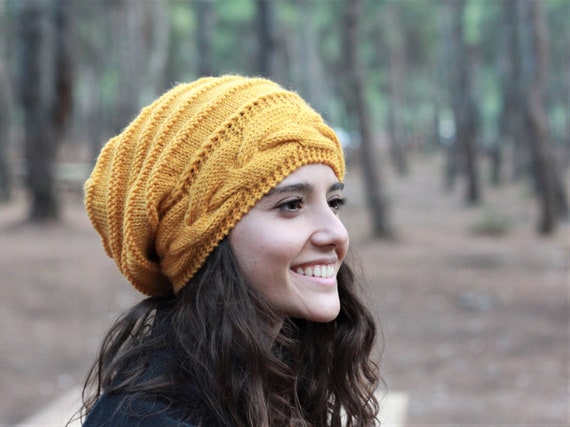In this photograph, we see a side view of a girl, likely in her late teens or early 20s, standing in an outdoor, wooded setting. She has medium-length, wavy brown hair cascading below her shoulders and is adorned with a mustard-yellow knit beanie. Her expressive dark brown eyebrows and long eyelashes frame her eyes, which are fully open and vibrant. She is smiling broadly, revealing her white teeth, and exudes an air of grace and elegance. Draped over her shoulder is a dark blue cloth. The background features a blurred mix of brown ground and several trees with brown trunks and sparse green leaves, contributing to the serene, natural atmosphere. The photograph is rectangular in shape and taken in landscape orientation.